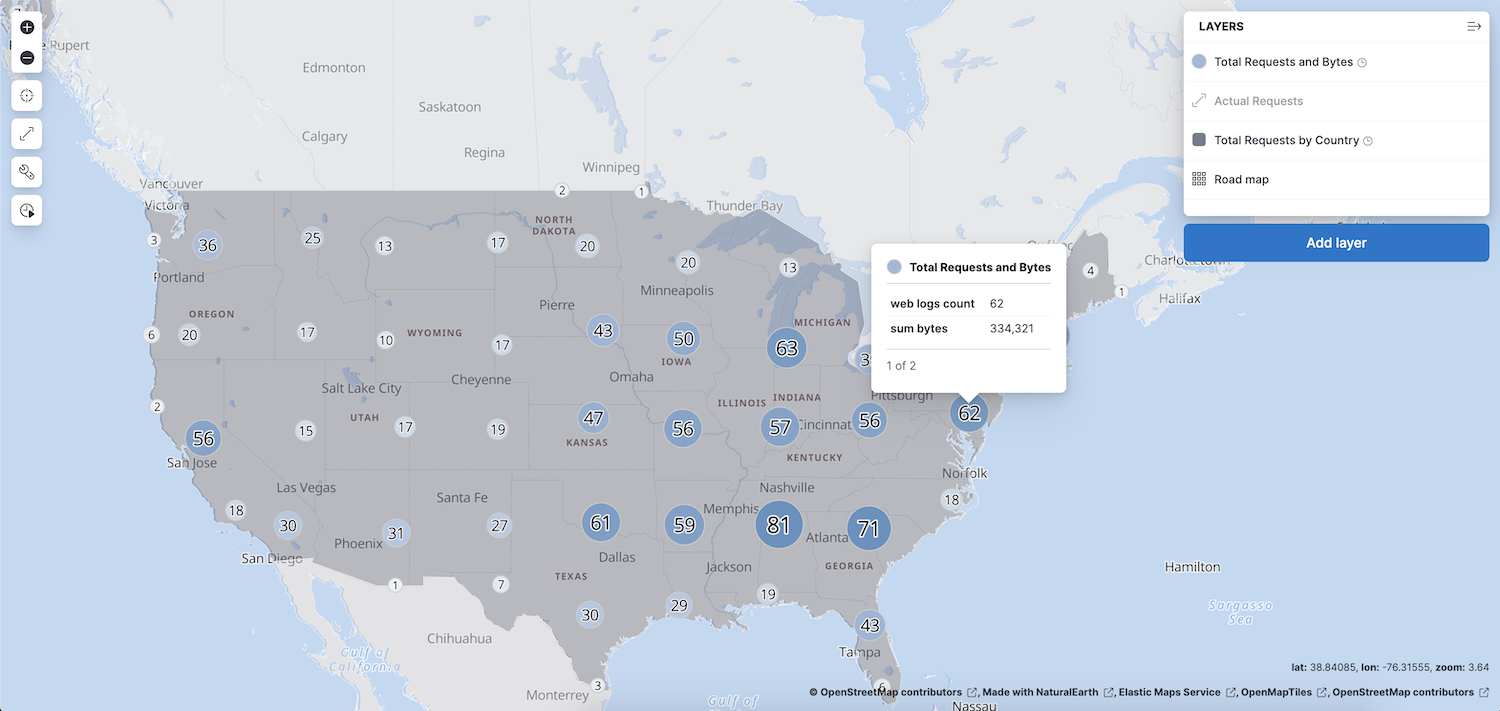This detailed map of the United States is shown in grey, with Canada and Mexico in a lighter grey above and below the U.S., respectively. To the right of the map is a key labeled "Layers," which includes options such as "Total Requests in Bytes," "Actual Requests," "Total Requests by Country," and "Roadmap." Additional options to "Add Layer" are also available. Below this key, the map data shows "Total Requests in Bytes" with a "Web Log Counts: 62" and "Sum Bytes: 334,321," indicating this is page 1 of 2. On the left side of the map, another key displays numbers assigned to each state in a seemingly random order. These numbers are highlighted in varying colors—some in blue, some in lighter blue, and others in grey—visually distinguishing different data sets or categories.